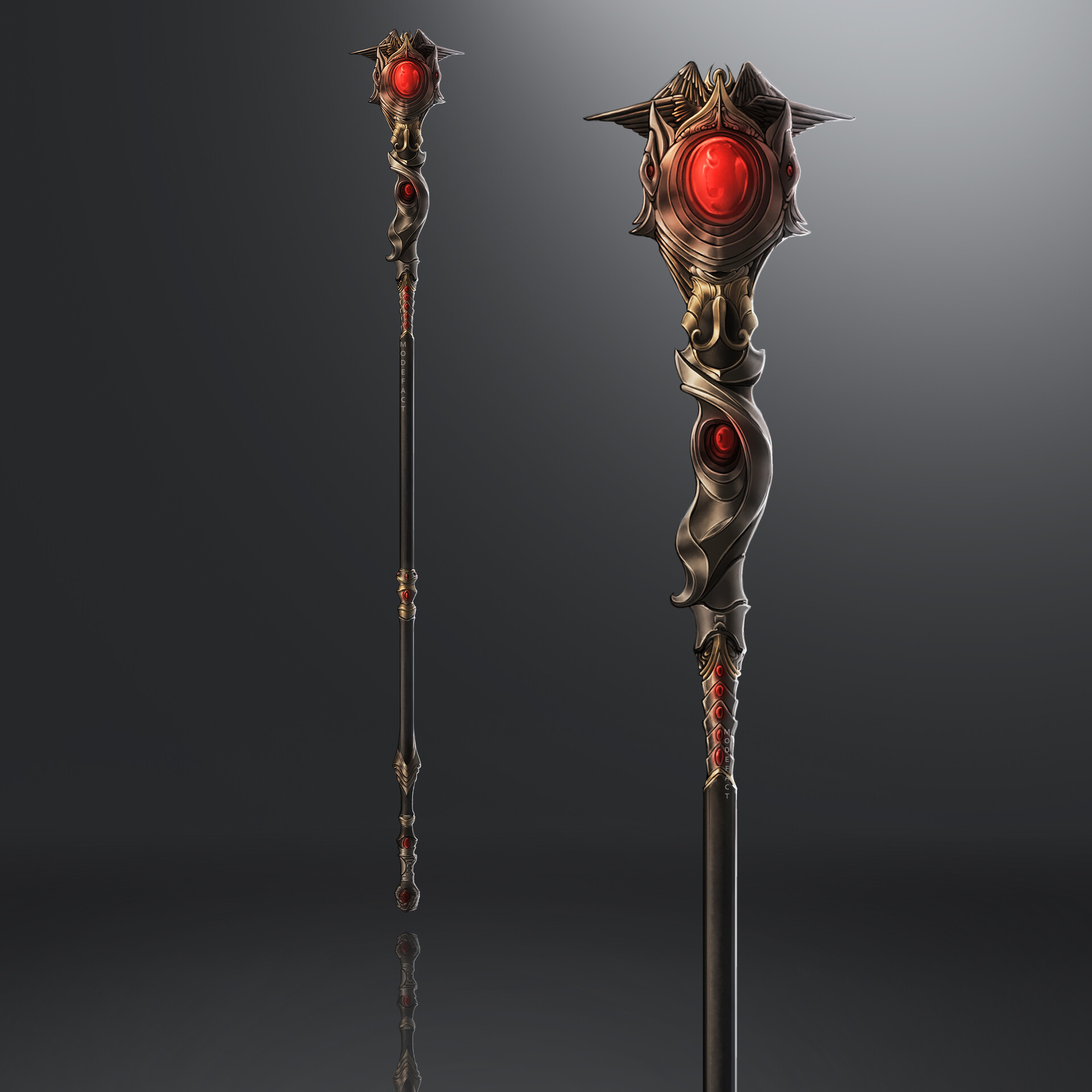This is an illustration featuring two ornate, mythical-looking scepters set against a dark gray background that transitions to a brighter, white section in the top right corner. Both scepters are detailed with intricate, swirling metal designs. The left side displays the entire length of one scepter, characterized by a prominent red, glowing gem at its top and resembling a dragon's eye just below it. The stick seems to be wooden with segmented parts. On the right, there is a close-up of the top portion of the other scepter, emphasizing the same glowing red gem. The overall composition accentuates the fantastical, dragon-like theme of the scepters, with their rich detailing and luminous gems.